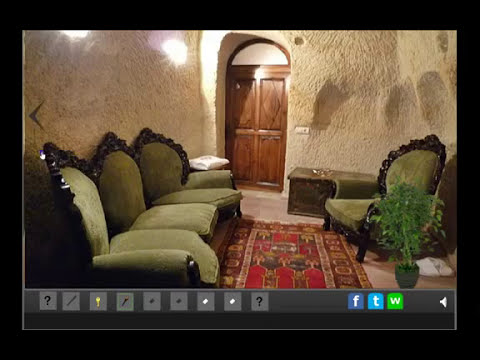The image depicts a room with beige, rough-textured stone walls that have an uneven surface. Dominating the far end of the room is a rich brown wooden door with an arched top, framed in white. To the right of the room, against the wall, are three green cushioned chairs, which appear to be upholstered in an olive green cloth or velvet fabric with dark wooden frames that offer a striking contrast. Another matching green chair is positioned against a white door on the same wall. Between these chairs, there is a rectangular brown rock with intricate patterns, featuring a red and yellow patterned rectangle in its center. The floor is adorned with a red rug that has gold accents and repetitive designs. Adding a touch of freshness, a small potted plant with vibrant green leaves is situated in the bottom right-hand corner, bringing a natural element into the room. The overall scene is seemingly taken from a screenshot on a computer program or a tablet, complete with a black border, various icons at the bottom, and social media icons on the right side.